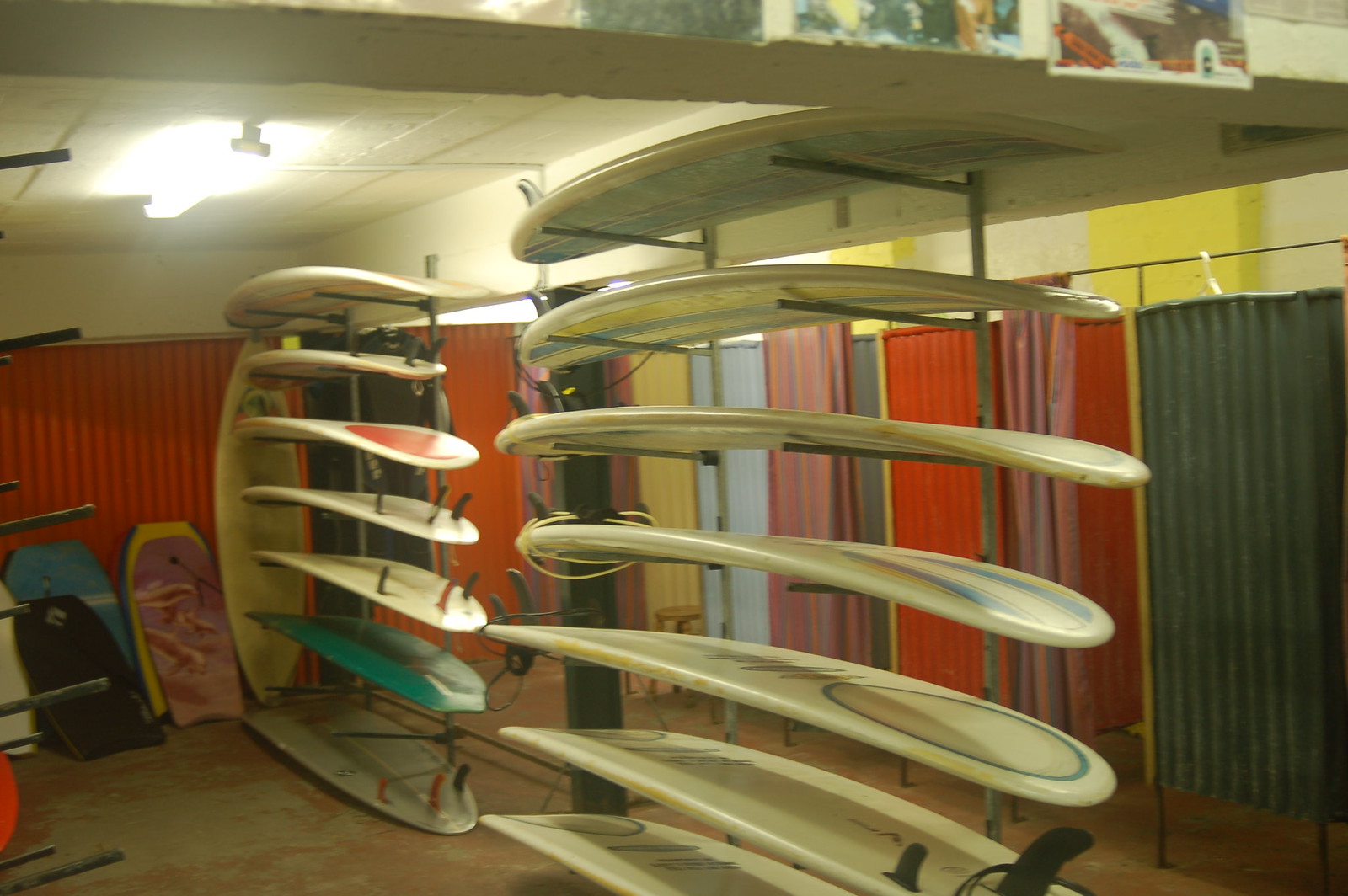The image depicts the interior of a surfboard shop with a somewhat industrial and confined atmosphere. The space features low ceilings with white styrofoam panels and a long halogen lamp suspended from above, suggesting the commercial nature of the building. Dominating the area are two steel racks supporting over a dozen surfboards, predominantly white, but there are also a turquoise board and one with a prominent red circle. These racks are front and center, with surfboards stacked neatly on top of one another. The room is partitioned by multicolored curtains reminiscent of hospital dividers, with hues of red, blue, and pink partially obstructing the view of the surfboards. Against the left wall, there is a striking red section, and the bright illumination of the room brings out the varied colors of the concrete floor, primarily featuring white with pink splotches. Additional colorful items, in blue and purple tones, are situated at the lower left edge of the image, although their purpose is unclear.